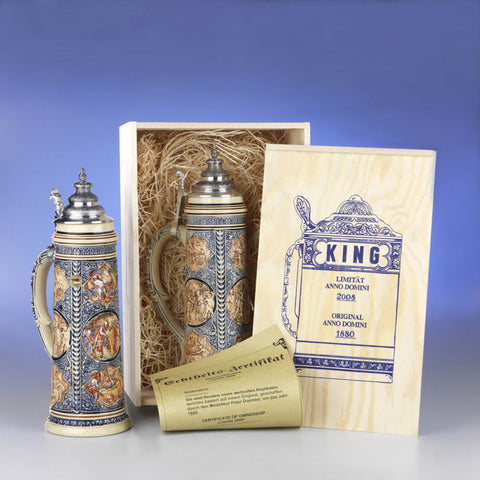This image depicts a beautifully crafted, tall porcelain beer stein adorned with an ornate metal cap. The stein features intricate blue scrolling flourishes that extend up its handle and frame multiple circular scenes depicting human figures. The background of the stein is a light tan or cream color, resembling natural clay. 

In the image, we see the stein twice. On the left, it stands on a shiny white table fading into a blue backdrop. In the center, the same stein is displayed inside an unfinished pine crate with its lid propped open. The interior of the crate is lined with dry straw for protection and includes a drooping olive-colored certificate. The lid of the crate is stamped in blue ink with an illustration of the stein, alongside text that reads, "King," "Original Anno Domini 1880," and "1650." 

The stein's picturesque details and collectible presentation suggest it could be an item of historical and artistic significance, potentially classified as fine china.